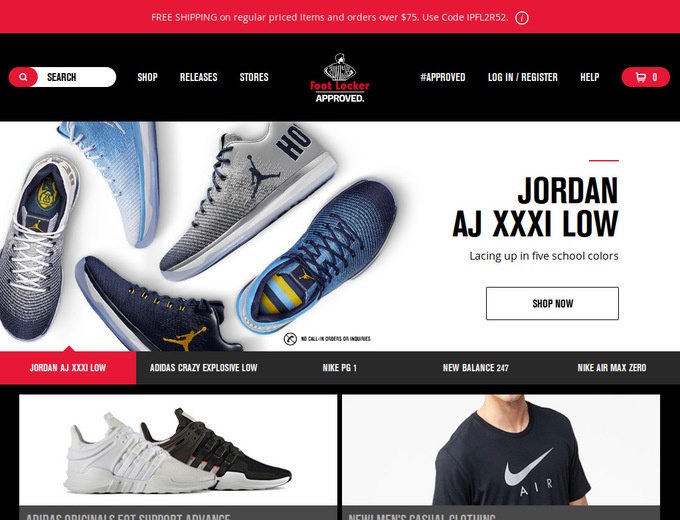At the top of the image, a long red rectangle features white text that reads "Free shipping on regular-priced items and orders over $75. Use code IPEL2852." Beneath it, a black rectangle contains a search bar with the placeholder text "Search." To the right, tabs labeled "Shop," "Releases," and "Stores" are displayed.

In the center, in smaller red text, the underlined name "Foot Locker" is seen, with the word "approved" underneath it. Above "Foot Locker" is an image of a referee wearing a black and white striped shirt. To the right, there are links labeled "#approved," "Login / Register," and "Help," followed by a red circle icon with a shopping cart inside.

Directly below this, there are images of various Jordan tennis shoes. One shoe is light gray with a black silhouette of a player reaching up to grab a ball. Below this are a set of blue shoes, and to the left, another blue shoe, followed by a dark blue shoe featuring the image of a yellow basketball player jumping up for a ball. To the right, text reads "Jordan AJ XXXI Low, lacing up in five school colors," next to a rectangle button that says "Shop Now."